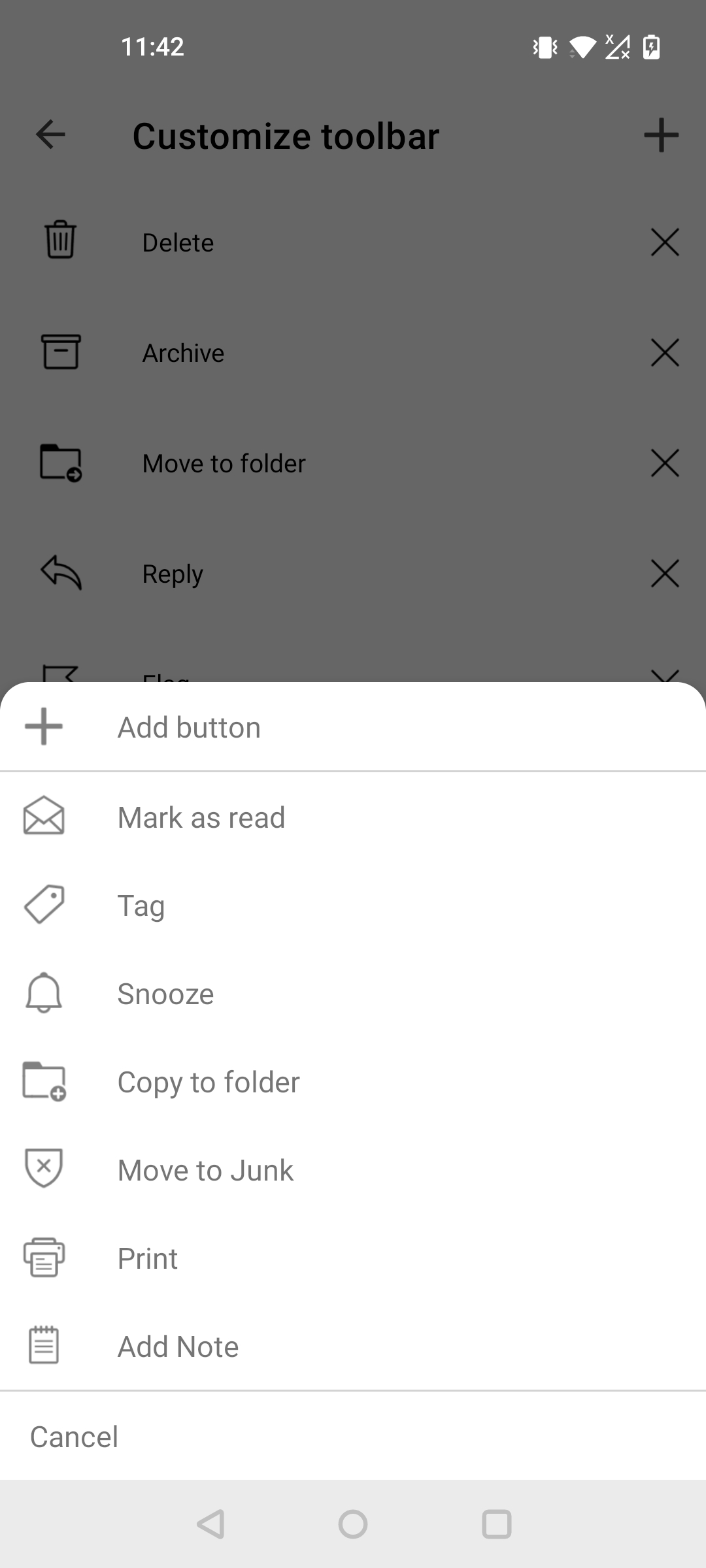This image, captured from a cell phone screen, shows a predominantly gray overlay at the top part of the screen enhanced by a white pop-up box. The white box features a series of icons and corresponding text labels. At the top, the phrase "Customized Toolbar" is visible within the gray area, followed by multiple icons and functions.

Inside the white box:
- A 'plus' icon labeled "Add Button"
- An envelope icon labeled "Mark as Read"
- A price tag icon labeled "Tag"
- A bell icon labeled "Snooze"
- An envelope with a tab icon labeled "Copy to Folder"
- A shield shape with an 'X' icon labeled "Move to Junk"
- A printer icon labeled "Print"
- A paper icon labeled "Add Note"

Under these icons, there is a faint gray line, the label "Cancel" is seen, and another faint gray line runs horizontally in the area beneath the "Add Button."

Additionally, in the gray area above the white box, several more icons with labels are present:
- A trash can icon labeled "Delete"
- A rectangle icon labeled "Archive"
- A folder icon labeled "Move to Folder"
- An arrow icon labeled "Reply" 

The overall white box seems to be a feature for customizing the toolbar on the screen.